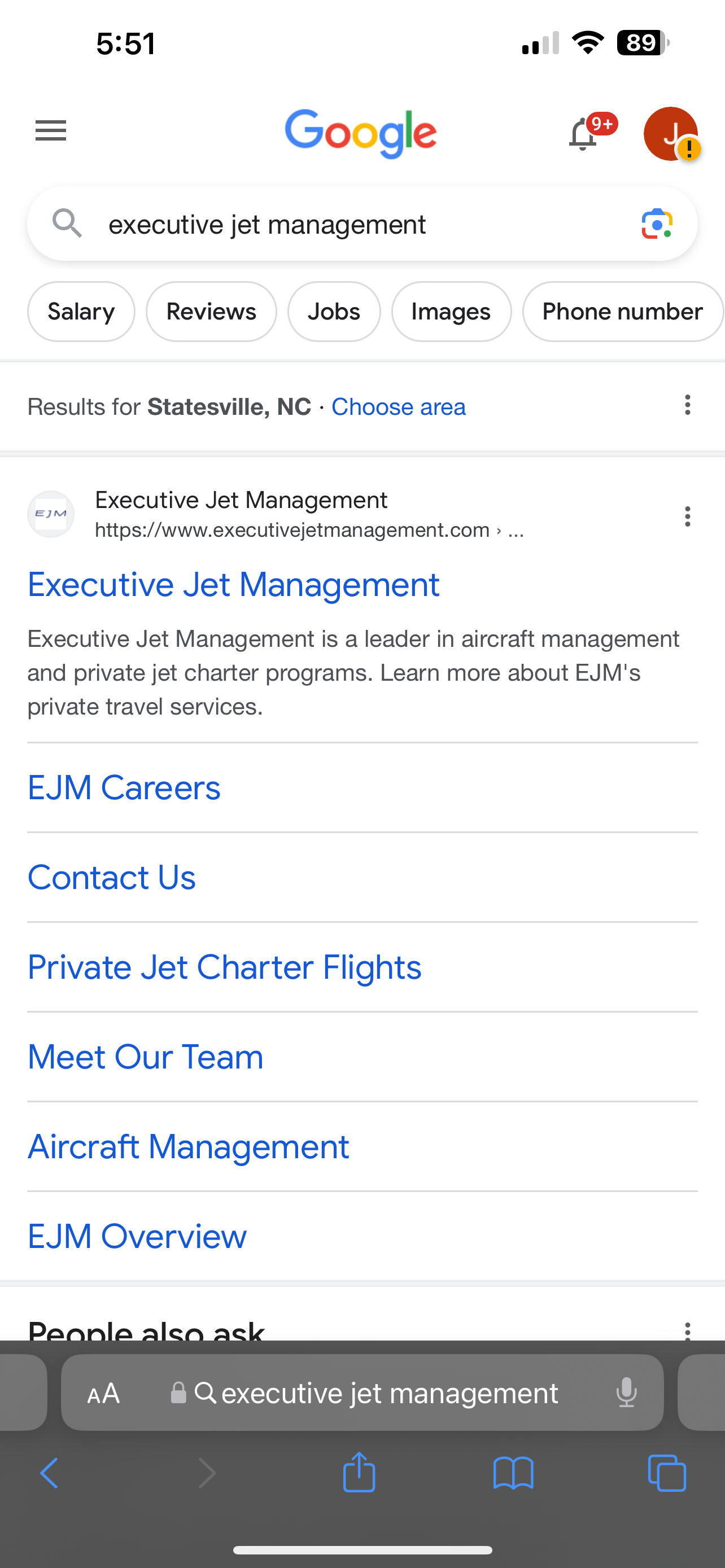A detailed caption for this image could be:

"The image shows a close-up of a smartphone displaying a Google search result page for 'Executive Jet Management'. At the top, the iconic multicolored Google logo is prominently visible above the search query. Below the search bar, clickable circular icons labeled 'Salary,' 'Reviews,' 'Jobs,' 'Images,' and 'Phone Number' are displayed. The location 'Statesville, North Carolina' appears just beneath these icons, accompanied by a blue link labeled 'Choose area' for selecting a different location. The main search result highlights the official website, 'executivejetmanagement.com,' with a brief description stating, 'Executive Jet Management is a leader in aircraft management and private jet charter programs. Learn more about EJM's private travel services.' Scrolling down, blue-font links such as 'EJM Careers,' 'Contact Us,' 'Private Jet Charter Flights,' 'Meet Our Team,' 'Aircraft Management,' and 'EJM Overview' are visible before transitioning to the black-font section labeled 'People also ask.' The bottom edge of the smartphone can also be seen in the image."